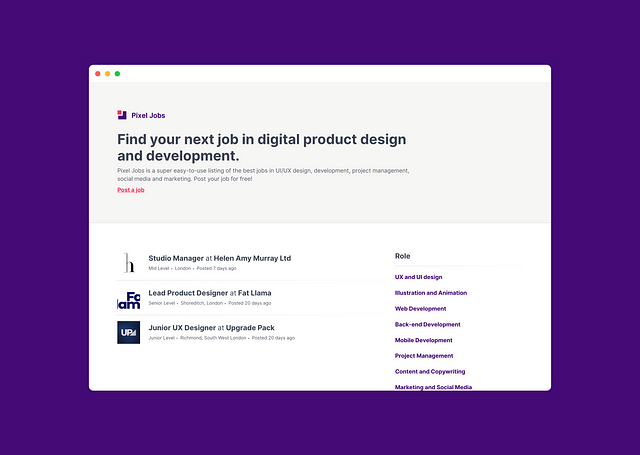The image in question is a digital graphic, approximately 30% wider than it is tall, framed by a dark purple border that occupies around 15% of the image's height and width on all sides. Within this border, there's a window designed to resemble a Mac operating system interface, identifiable by the three dots—red, yellow, and green—in the upper left corner.

The top portion of the window, roughly the next 45% of the screen's height, features a light gray background overlaid with text. The header on the left side reads "Pixel Jobs," accompanied by a logo consisting of a red square merged with a blue square. Below this header, in large, bold black font, is the prominent message: "Find your next job in digital product design and development." Beneath this tagline, two lines of smaller, less legible text are present, followed by the phrase "Post a job" in red text, which is underlined.

Transitioning into the lower half of the window, the background shifts to white, showcasing three job titles aligned on the left side: "Studio Manager," "Lead Product Designer," and "Junior UX Designer."